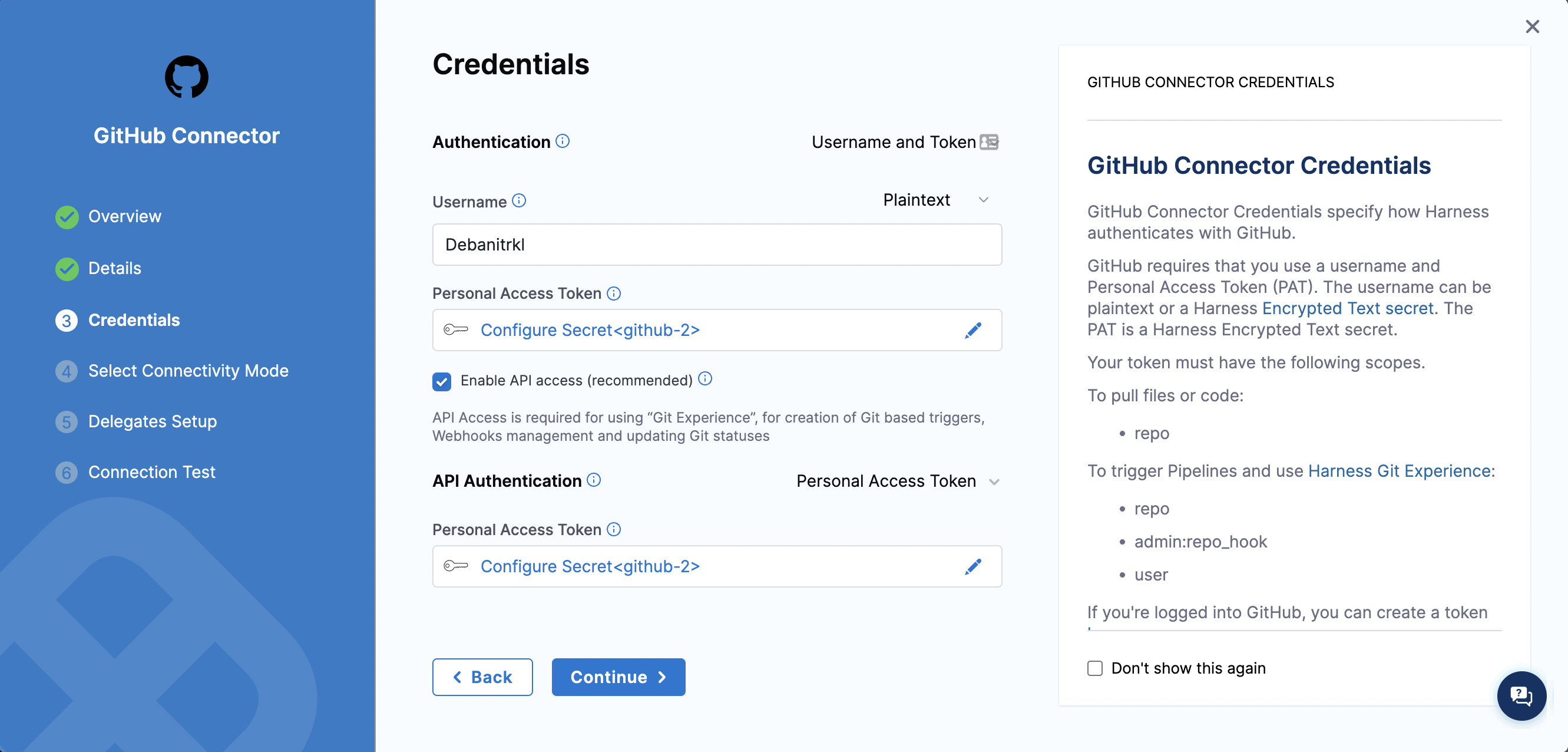Screenshot of a webpage with a predominantly white background. On the left side, there's a vertical blue rectangle featuring a layout of various icons and labels. At the top of this blue section, there's a small black circle containing a blue silhouette of a cat head. Directly beneath the circle, "GitHub Connector" is written in white font.

The blue rectangle features a vertical list of menu items also in white font: Overview, Details, Credentials, Select Connectivity Mode, Delegate Setup, and Connection Test. Icons indicating status are also present: a green circle with a checkmark next to Overview and Details, and a white circle with the number "3" next to Credentials, indicating the active menu section.

On the right side of the blue rectangle, the Credentials menu is displayed against a white background with black text. At the top, the heading "Credentials" is followed by sub-sections including "Authentication," "Username," and "Token." Under "Username," there is a field that contains the text "Debantrid". Further down, under "Personal Access Token," there is another field displaying "Configure Secret GitHub 2" in blue font. Below these fields, an option labeled "Enable API Access" is also visible.